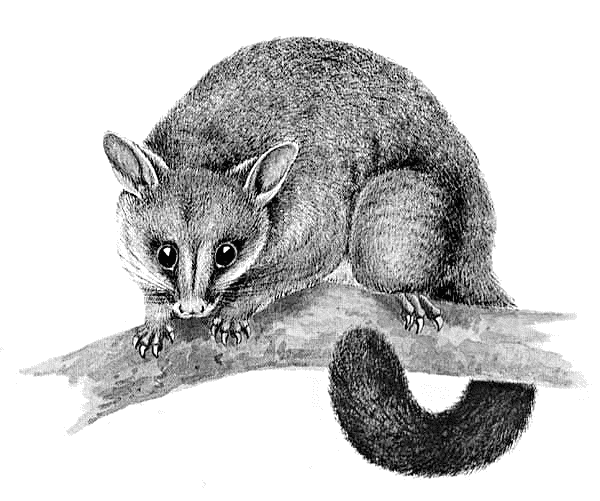This black and white illustration features a detailed animal perched on a large, textured tree branch that extends from the right side of the image, bending downward to the left. The background is a stark white, offering no additional context or scenery. The animal, which has a dense, fluffy coat and a long, bushy tail that curls around underneath the branch, resembles a small mammal, possibly a mixture of a fox and a raccoon. Its head, which is pointed with rounded ears and big black eyes, is turned down as it looks towards the viewer. The animal's front paws, each equipped with tiny claws, grip the branch tightly, while its rear left paw is also visible. The illustration utilizes black pencil, charcoal, or ink, giving the drawing a grayscale effect, while the branch appears almost watercolor-like. Despite the amateur perspective, the artist has put remarkable effort into capturing the texture of the fur and the details in the claws and eyes, resulting in an image that feels dense and lifelike, yet distinctly a drawing.